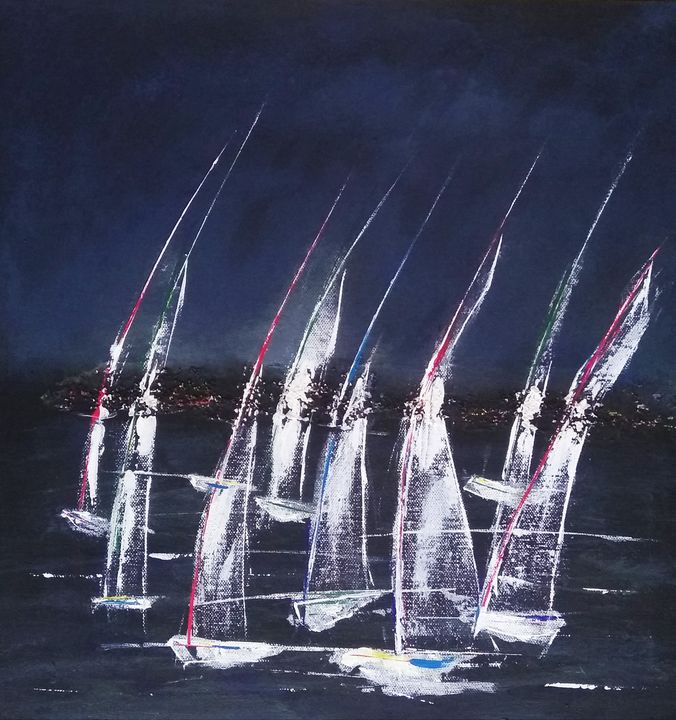This painting, displayed on a slightly rectangular canvas, showcases a nighttime maritime scene rendered in abstract style. The entire background is enveloped in deep, varying shades of dark blue, from the sky to the ocean below. The horizon features a distant pier or skyline, faintly lit and silhouetted against the night sky. The focal point of the artwork is eight minimally detailed, white sailboats scattered across the ocean. Each sailboat is crafted with quick brush strokes, emphasizing their small, singular masts and sails. Some boats exhibit subtle color highlights, with dark pink and blue accents on the masts. The motion of the sailboats is suggested by white lines in the water, enhancing the sensation of movement on the dark, tranquil sea.